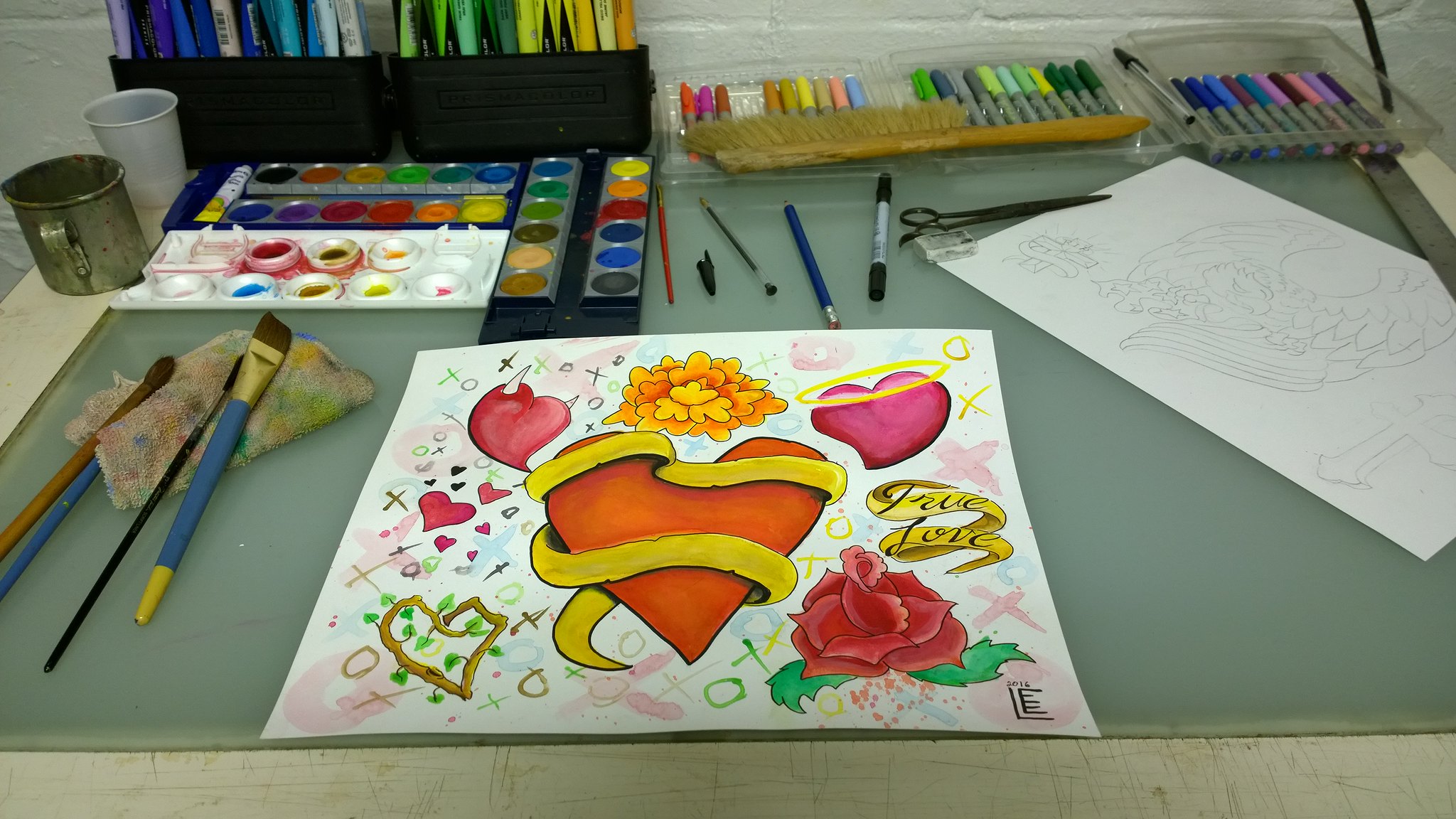The photograph captures an artist's workspace taken at a slight angle, looking down on a rectangular gray table bordered by a white edge. Centered on this table is a white sheet of paper showcasing various tattoo-style illustrations, predominantly hearts and flowers. The standout drawing is a red cartoon heart with a banner wrapped around it. To the upper left, there's a heart with white horns, and to the upper right, a heart with a halo. Below these motifs, a gold banner elegantly displays "true love" written in cursive, accompanied by a side-profile rose and a heart made of sticks.

On the right side of the table is another sketch, uncolored, on a white rectangular piece of paper. Nearby, a collection of paintbrushes, with blue and black handles, lie on a paint-smeared rag. Adjacent to the brushes are neat trays of watercolor paints.

Further to the right edge of the table, there is a proportional and organized collection of colored pens and markers. Behind this workspace, against a white brick wall, more markers are lined up. A metal cup and a plastic cup are also visible, adding to the artistic clutter that defines this vibrant and creative space.